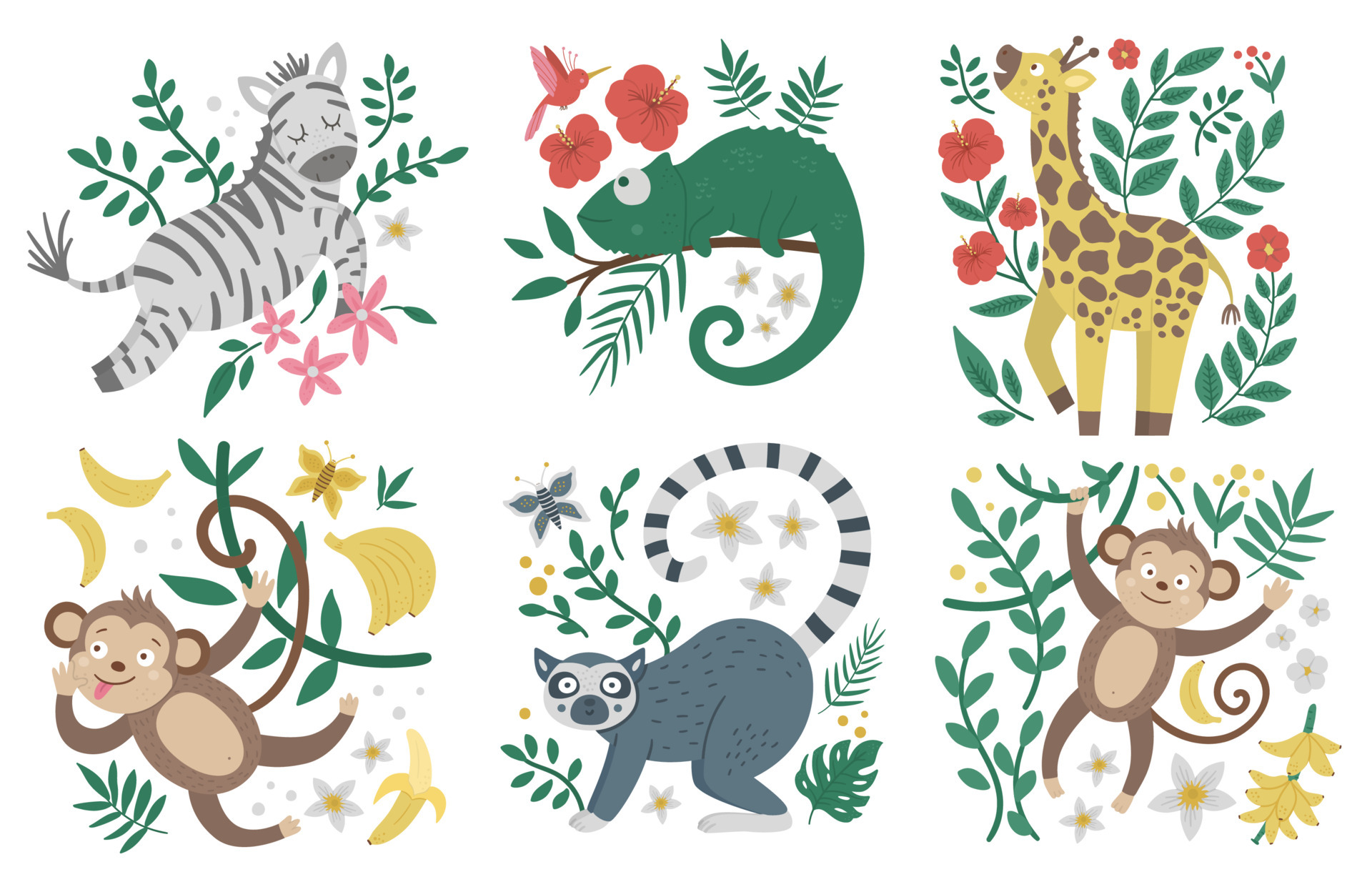This image is a collection of six minimalistic, 2D illustrations of different animals, arranged in a grid with two rows and three columns. The designs are cute, comic-style, and have minimal texture. Each illustration features natural elements like flowers and leaves. Starting from the top left, the first illustration is of a gleefullly prancing zebra surrounded by red and pink flowers. To the right, the second illustration shows a chameleon perched on a tree branch among red flowers. The top right illustration depicts a happy giraffe looking up amidst red flowers and green leaves. In the bottom row, the leftmost picture shows a monkey hanging from a vine with bananas and pink flowers. The central illustration in the bottom row features a lemur accompanied by a yellow butterfly and bananas. Finally, the bottom right image portrays another monkey hanging from a vine, surrounded by white flowers, green leaves, and bananas. The background uses a palette of gray, green, pink, yellow, brown, and blue-gray tones to create a seamless, joyful atmosphere.